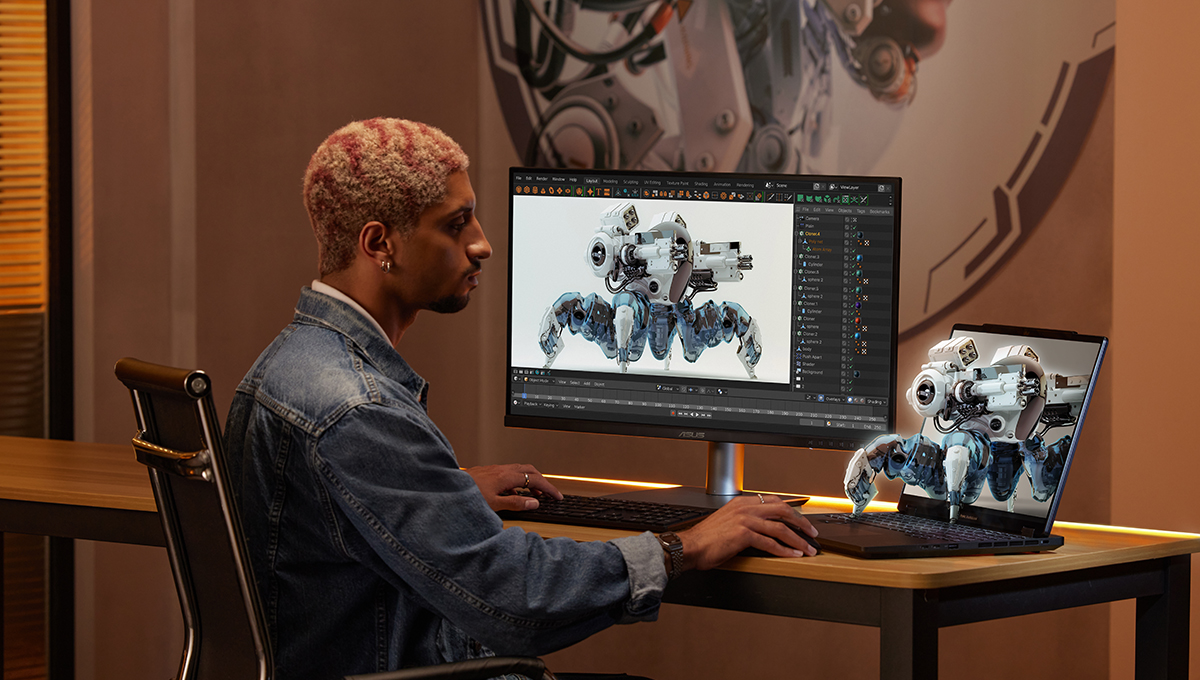This captivating photorealistic image captures a young African American man with rich brown skin, seated in a black leather desk chair with a handle at the back. His striking hair, a blend of blonde and burgundy stripes, highlights his artistic flair. He sports a denim jacket, a watch, and two small silver earrings in his right ear. His meticulously groomed facial hair includes a slight beard and mustache. The scene is set in a modern, highly graphic room, featuring a desk with a light wood top and a darker base.

In front of him, there is a full-size black monitor displaying a white and blue robotic creature, which he has meticulously designed. To his right is an open laptop, from which the same robot appears to be emerging, giving an impression of it coming to life directly from the screen. This imaginative detail, akin to a step above 3D printing, underscores his deep engagement with robotics and graphic design. His left hand is on the keyboard connected to the desktop monitor, while his right hand touches the laptop, emphasizing his control over the digital and seemingly physical creation. Adding to the modern aesthetic, the backdrop features a partial view of a large disk on the wall, further enhancing the visual allure of the room.